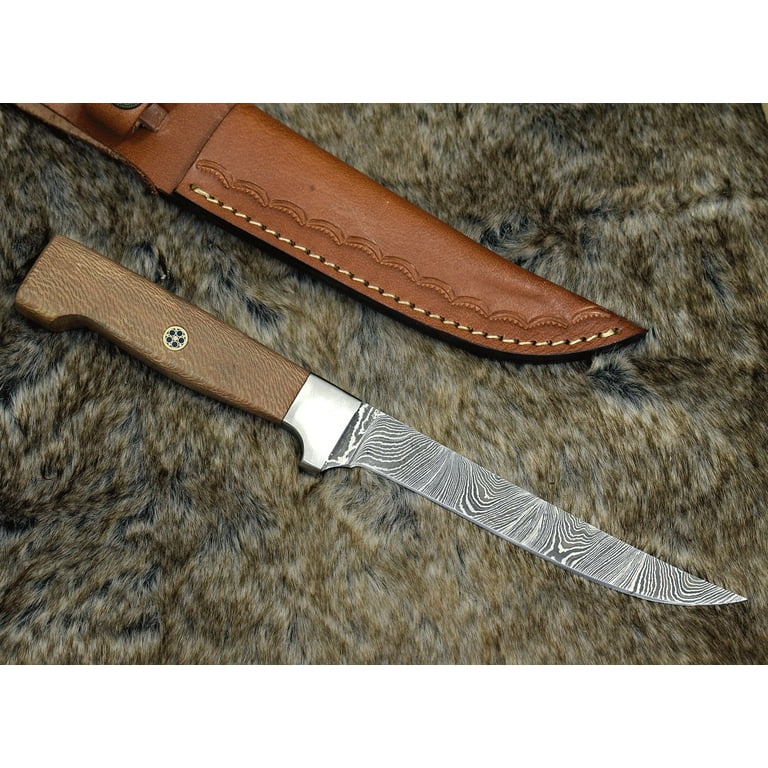This full-color, square photograph depicts a beautifully crafted knife and its leather sheath, artfully arranged on what appears to be a fur rug. The background comprises soft, light brown fur with darker black patches and hints of white, creating a rich, textured backdrop. The sheath, which occupies the upper left corner and extends diagonally to the right middle of the image, is made of dark brown leather and features intricate gold stitching and a decorative pattern. 

The knife, positioned below the sheath, boasts a finely polished wooden hilt with a light brown finish and an emblem resembling a Texas star, gold with black accents, embedded into it. The blade itself is a striking mix of black and silver hues, reminiscent of the swirling patterns seen in Damascus steel, creating an almost fingerprint-like appearance. The overall presentation suggests a deliberate, high-quality showcase, perhaps intended for sale or display. The expert craftsmanship of both the sheath and the blade, along with their careful positioning against the luxurious fur, highlights their aesthetic and functional appeal.